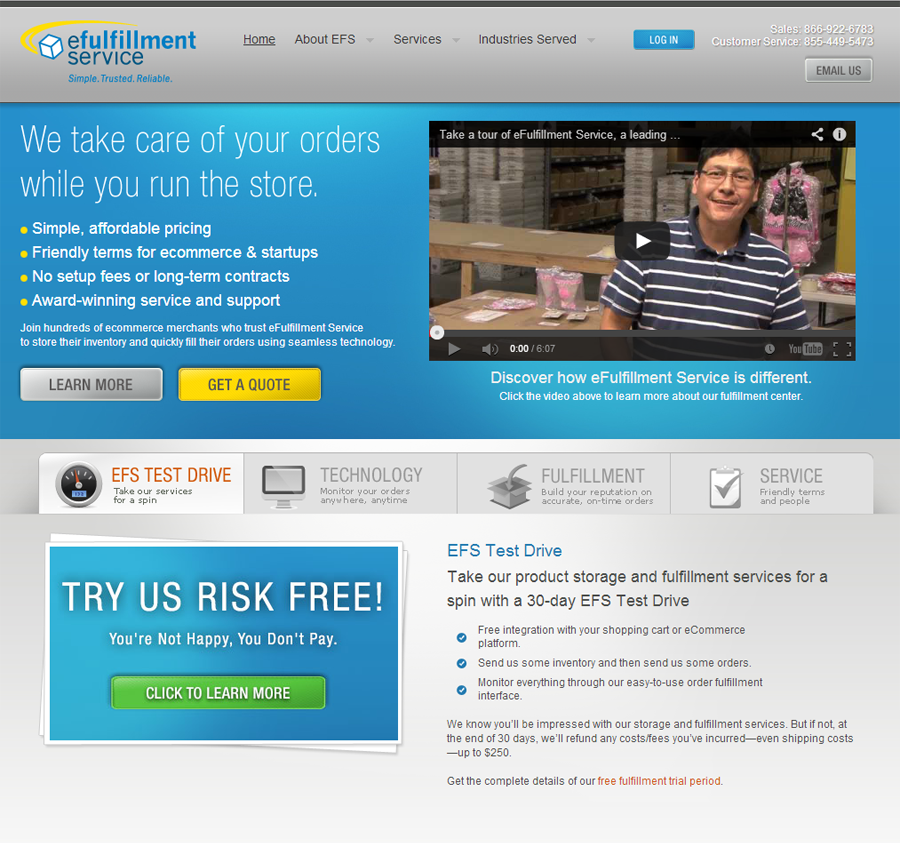A detailed descriptive caption of the photographed web page:

The web page features a predominantly gray, blue, white, yellow, and green color scheme. At the top of the page, there is a gray banner. Below the banner, a white cube outlined in blue is prominently displayed. Encircling the cube is a yellow banner that reads "E-fulfillment service" along with the words "single," "trusted," and "reliable" in blue. The navigation tabs positioned nearby include "Home," "About EFS," "Services," and "Industries Served."

In the upper right corner, there is a blue "Log In" button. Contact information is provided with a phone number for sales, a phone number for customer service, and a gray "Email Us" button. Below the top banner, a blue banner contains white text stating, "We take care of your orders while you run the store." 

A series of yellow bullet points are listed beneath this banner highlighting key features of the service: "Simple affordable pricing," "Friendly terms for e-commerce and startups," "No set-up fees or long-term contracts," and "Award-winning service and support." Adjacent to these bullet points are two action buttons: a gray "Learn More" button and a yellow "Get a Quote" button.

The web page also features a video thumbnail showing a man smiling, wearing glasses, and a striped polo shirt, standing in what appears to be a warehouse setting. The caption under the video states, "Take a tour of the E-fulfillment service." 

A notable blue rectangle banner includes an inviting proposition in large font, "Try us, risk-free." The accompanying text in white reads, "You're not happy, you don't pay." At the bottom of the page, a green button is prominently displayed with the call-to-action, "Click here to learn more."

This detailed layout and organization of web page elements reflect a comprehensive e-fulfillment service's customer engagement and support offerings.